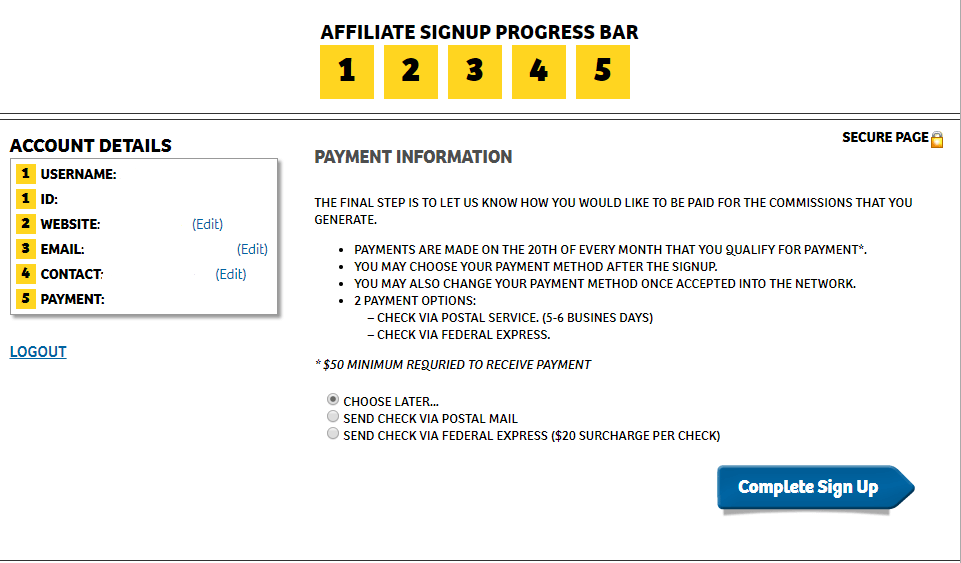The image illustrates the affiliate signup process in a structured and detailed manner. At the top, there's a progress bar highlighting the different stages of registration. Below it, a yellow box with black writing numbers 1 through 5 is displayed. On the left side of the page, there is a section for account details, listing fields in vertical order: username, ID, website, email, contact, and payment.

In the middle section, the focus shifts to payment information. It explains the process for submitting payment details and securing your account, indicated by a "secure page" label accompanied by a lock icon on the far right. The text beneath the payment information outlines the final step, stating, "The final step is to let us know how you would like to be paid for the commissions that you generate."

To the far right, a clear instruction is given regarding the $50 minimum requirement to receive payment. Below this, there are three checkbox options for payment methods: 

1. Choose later (this option is currently selected)
2. Send check via post mail
3. Send check via Federal Express with a $20 surcharge per check

On the extreme left, in blue writing, there is a "Log Out" icon for users to exit the process if needed.